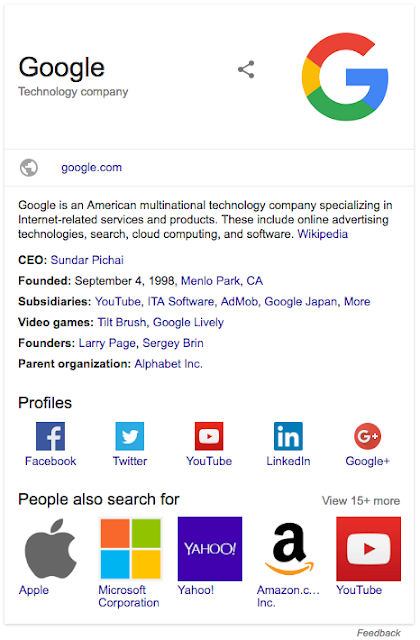The image is a detailed screenshot showcasing the right-hand side panel of a Google search results page, likely the result of searching for "Google." The central focus is the prominent Google logo - a multicolored 'G' in red, yellow, green, and blue hues. Below the logo, Google is labeled as a "Technology Company," with a direct link to Google.com provided.

Further down, the panel offers a concise description originating from Wikipedia, identifying Google as an American multinational technology company specializing in internet-related services and products. It highlights areas such as online advertising technologies, search, cloud computing, and software development, including a link to the full Wikipedia page for additional information.

The panel also features key details about the company:  
- **CEO:** Sundar Pichai  
- **Founded:** September 4, 1998, in Menlo Park, California  
- **Subsidiaries:** including YouTube, ITA Software, AdMob, and Google Japan, with a "more" option indicating additional subsidiaries  
- **Video Games:** Tilt Brush, Google Lively  
- **Founders:** Larry Page and Sergey Brin  
- **Parent Organization:** Alphabet Inc.  

Moreover, the panel lists Google's profiles on various social media platforms such as Facebook, Twitter, YouTube, LinkedIn, and the now-defunct Google Plus. It concludes with a section titled "People also search for," suggesting other technology giants like Apple, Microsoft Corporation, Yahoo, Amazon.com, Inc., and YouTube as related search interests.